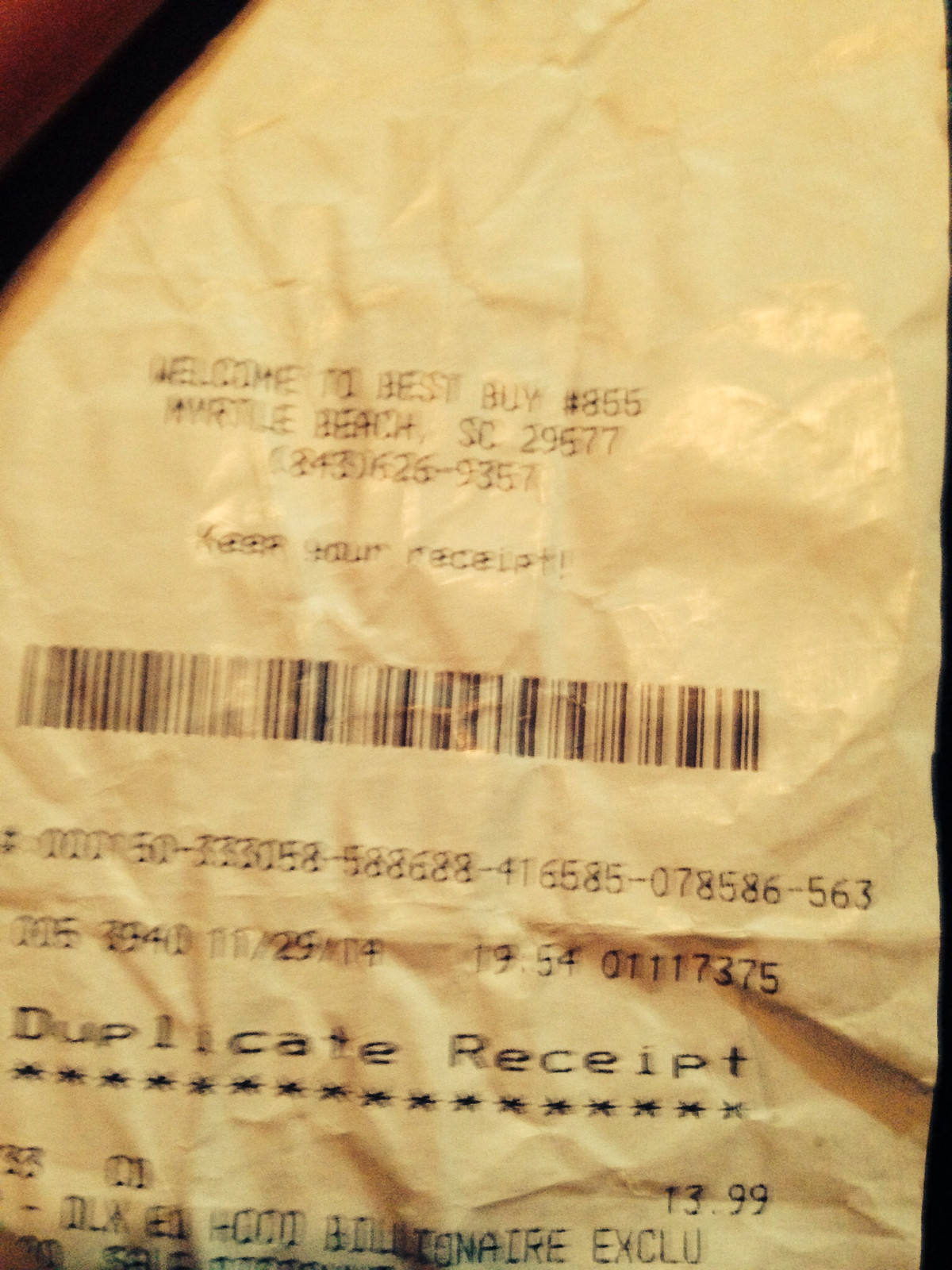The image depicts a receipt with a distinct yellowish tint, likely due to the lighting or age of the paper. Prominently featured is a barcode and the wording "Duplicate Receipt." At the top, it reads "Welcome to Best Buy," followed by the store number "885" and the location "Myrtle Beach, South Carolina." The receipt includes a reminder to "keep your receipt" along with various numerical details related to transactions or items purchased. The barcode and the plethora of numerical data capture important transactional information.